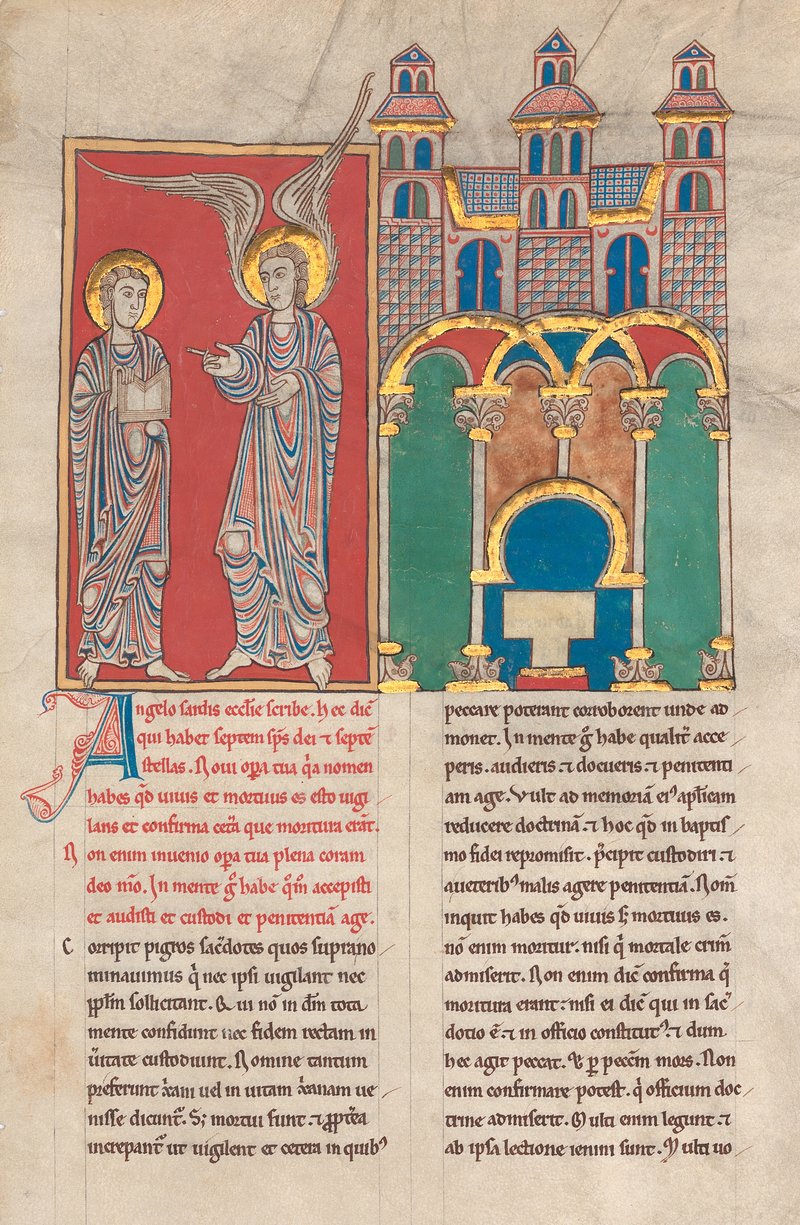This rectangular manuscript, approximately six inches high and four inches wide, likely originates from the European Medieval Period, as evidenced by its stylistic elements. The background has aged into an off-brown color, indicative of years of wear. The upper half of the manuscript features a vivid, colorful illustration. On the left side of the illustration are two figures: an angel with wings and another figure, possibly Jesus, cloaked in blue, red, and white robes with a halo behind his head. These figures appear to be interacting. Adjacent to them on the right is a detailed depiction of a medieval castle or temple rendered in blues, greens, browns, and golds. Beneath this illustration is a layer of Latin text, presented in a highly stylized cursive typical of Medieval manuscripts. The text is organized into two columns, with the initial paragraphs in red and the remaining text in black. The overall aesthetic of the manuscript is enhanced by its use of vibrant colors, including green, red, blue, and gold, lending it a poster-like appearance that captures a religious scenario with significant visual appeal.